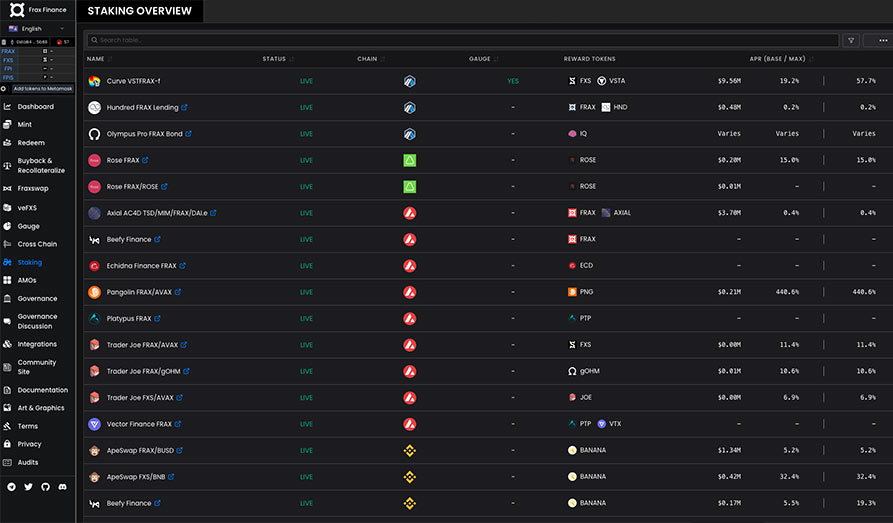The screenshot features a predominantly black background with a user interface that appears to be part of a gaming ranking site. The layout is organized into multiple columns within a large, central box, with a left sidebar featuring a vertical list of options. 

At the top-left corner of the interface, there is an indistinct logo resembling a circle within a square, although the accompanying text is unreadable. Adjacent to the logo, the title "Staking Overview" is prominently displayed in white text against the black backdrop.

The main content area displays eight distinct columns. The first column is labeled "Name" and includes various circular profile images, each accompanied by presumably the names of players. These profile images vary in color.

The second column features dark green values, although the specific label for this column is not clear. The third column contains a series of symbols: three round blue icons at the top, followed by two green squares, several red circles with white lightning bolt symbols, and three yellow symbols at the bottom.

Subsequent columns display various statistics related to the players’ gaming results, but the exact details are indistinguishable due to the small size of the text and icons. The overall layout suggests a detailed and organized interface designed for tracking and comparing player performance metrics.